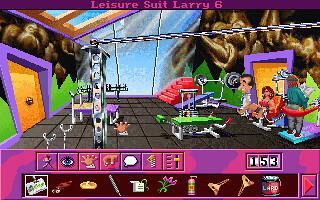This is a detailed screenshot of the computer game "Leisure Suit Larry 6," with the game's title displayed at the top in pinkish-red letters. The scene is set in a cartoonish gym featuring a tile floor and various workout equipment. Prominently, there is a weight bench with a barbell on a rack, and a slanted purple bench positioned for chest workouts. Additionally, there is a weight machine with a green cushion. The gym also includes a red stairway in the background, a brown door set in a purple doorframe on the left-hand side, and a wall with a mix of green jagged lower sections and brown rocky upper sections. The room is adorned with an irregular-shaped window or mural and skylights. On the right side of the image, several characters are standing in front of a door with a purple archway and golden-brown trim. The bottom of the screenshot showcases a purple and pink swirled toolbar displaying multiple game items and perhaps a score reading 153.